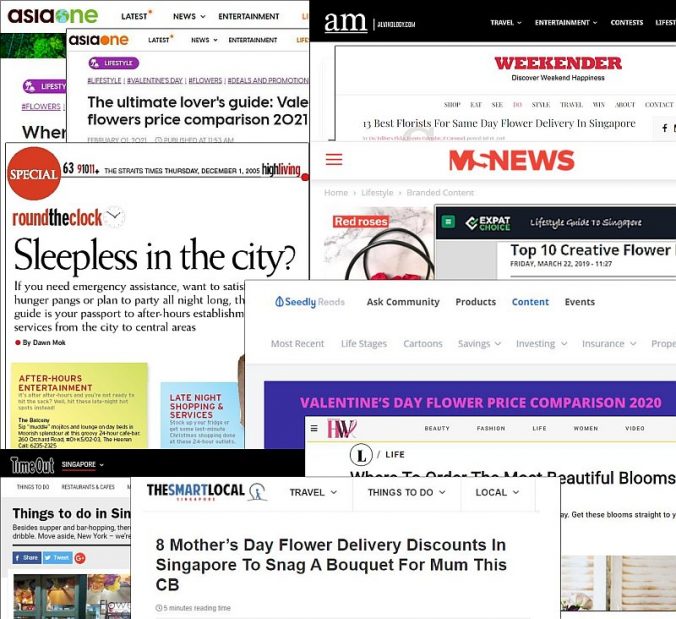This screenshot showcases a dynamic collage of ten overlapping images of various magazine websites. Each website front page's purpose and design are seen clearly despite the haphazard arrangement. In the top left corner, there are two images from "Asia 1," one of which displays an article titled "The Ultimate Lover's Guide for Price Comparison in 2021." Adjacent to these, on the right, is another website labeled "AM," punctuated by a distinct black bar at the top that indicates sections such as "Travel," "Entertainment," and "Contest." Below "AM" is the website "MS News," while to its left is a page titled "Round the Clock" with an article named "Sleepless in the City" at the upper section. The collage, though seemingly random in its layout, effectively captures the diversity of content and design across these magazine websites.